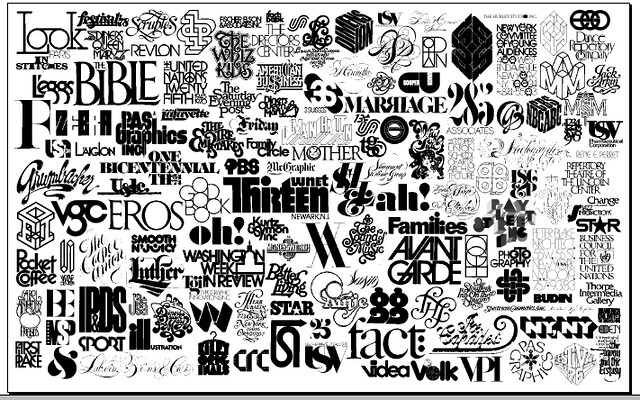The image is a black-and-white graphic design resembling an intricate collage of various logos, ads, and company names, with each element closely packed together. It features a diverse array of fonts and styles, resulting in a visually complex and textured composition. On a white background, the logos, primarily in black or grayscale, are haphazardly scattered across the image, without any overt pattern or alignment. Distinct phrases and logos can be identified, such as "13" prominently displayed at the center, "families" nearby, "avant-garde" below, and "fact" at the bottom center. Additional recognizable entities include "The Bible" at the top left, "First Place," "Star," "Better Living," "Revlon," "Legs," "New York, New York," and "The Sound of Music," among others. A black border frames the entire composition, defining the edges of this eclectic conglomeration of text and imagery.